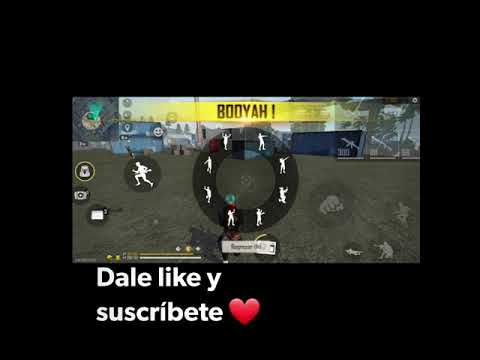This image appears to be a screenshot from a game that resembles Call of Duty, though it is extremely blurry and grainy. The image is framed by a thick black border, even thicker on the top and bottom. Prominently at the top of the image, a yellow banner with the word "Booyah!" in black, bold letters stands out. Below this, the central part of the image features a series of emotes that display various body movements, such as a person with arms raised or skipping, although it's difficult to discern the exact actions due to the blur.

The scene appears to be set outdoors, possibly in a back alley, evidenced by the presence of a large blue trash bin and a long trash container. The backdrop includes a building and a brown dirt road, adding to the urban setting. Adding to the ambiance, the soldiers and their equipment hint at the game's combat-oriented theme.

In the bottom left corner, white text reads "Dale Yeah, Like, Why, Subscript" accompanied by a red heart emoji, suggesting a prompt, likely in another language, encouraging viewers to subscribe to the content. The name of the game or channel seems to be indicated on a leaflet located at the bottom right of the image, though it's challenging to get the exact details due to the black background dominating much of the frame.